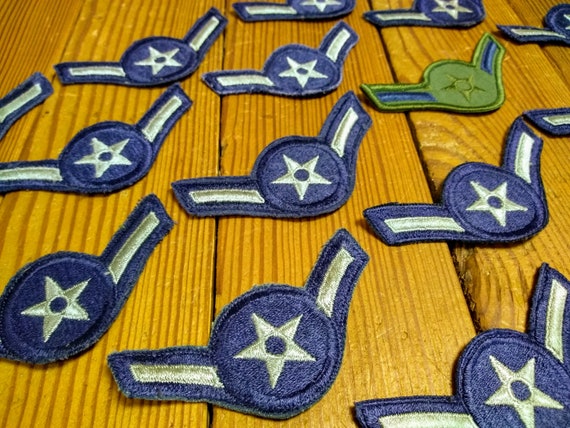The image features a collection of intricately embroidered patches resembling Captain America's iconic military-style emblem. Each patch showcases a blue circle with a central silver five-pointed star, flanked by blue wings that extend outwards on either side, adorned with silver bars. These patches, designed to be ironed onto clothing, are meticulously arranged on a caramel-colored wooden table, creating a visually appealing layout. There are a total of thirteen patches, most of which follow the same blue and white color scheme, except for one unique green patch situated on the right-hand side. This green patch mirrors the design but features a green circle and star with white bars instead of the traditional blue, adding a distinctive touch to the uniform collection. The wooden background's warm tones complement the vibrant hues of the embroidered patches, enhancing the overall aesthetic appeal of the scene.